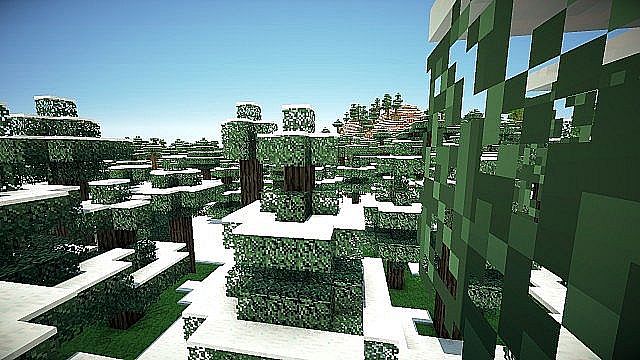This computer-generated image showcases a highly stylized, cubist representation of buildings and landscapes. Dominated by rectangular and square cubes, the scene presents a distinctive, blocky aesthetic. On the right-hand side, a series of stacked cubes form what appears to be a building's wall. The design gives a sense of terracing throughout the composition. Centrally located is another cubic building, interconnected by white walkways that traverse a gradient of green blocks, transitioning from dark to light green hues. On the left side, more white walkways guide the viewer through an arrangement of angular, block-style structures that recede into the distance. In the background, to the center-right, a small mountain rises, its left slope adorned with trees while the right side displays exposed brown rock features. The meticulously designed scene combines natural elements with geometric forms, creating a harmonious yet visually striking landscape.